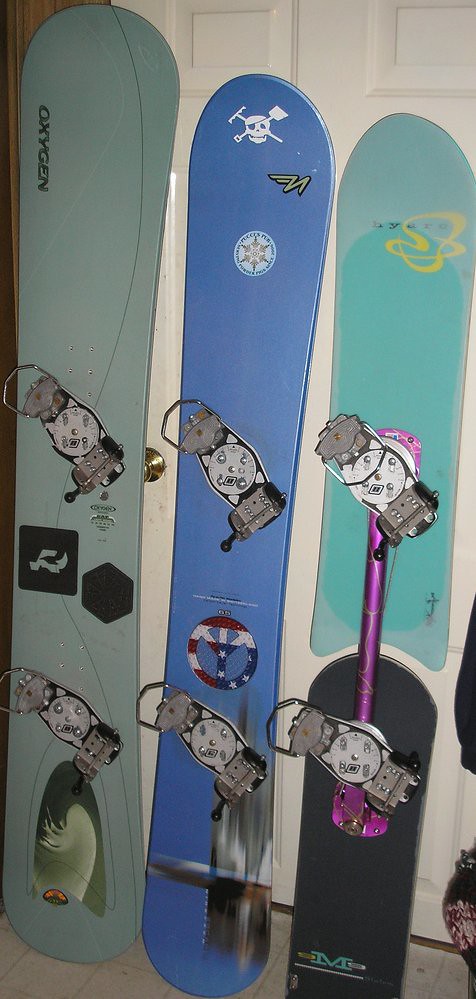This color photo displays a collection of three snowboards, each with unique designs and varying in size. The snowboard on the far left is the tallest and features a muted mint green or light grayish blue color, with the brand name "Oxygen" prominently displayed at the top in black lettering. It is equipped with grey and white bindings to secure special boots.

The middle snowboard, slightly shorter, is a bright blue color adorned with a white skull and crossbones design. Instead of crossbones, it has a rake and snow shovel. Below the skull, there is a grey and white peace sign decorated with American flag colors, red, white, and blue stars.

The shortest of the trio is the snowboard on the right, which is distinct in its design. The top section is an aqua blue color, while the bottom half is a dark gray or black. These two sections are connected by a striking purple or pink metallic rod. The bindings on this board are also grey and white.

Each snowboard has specialized bindings, suggesting the need for specific boots, and they are arranged in descending order of height from left to right, creating a visually appealing and detailed display.